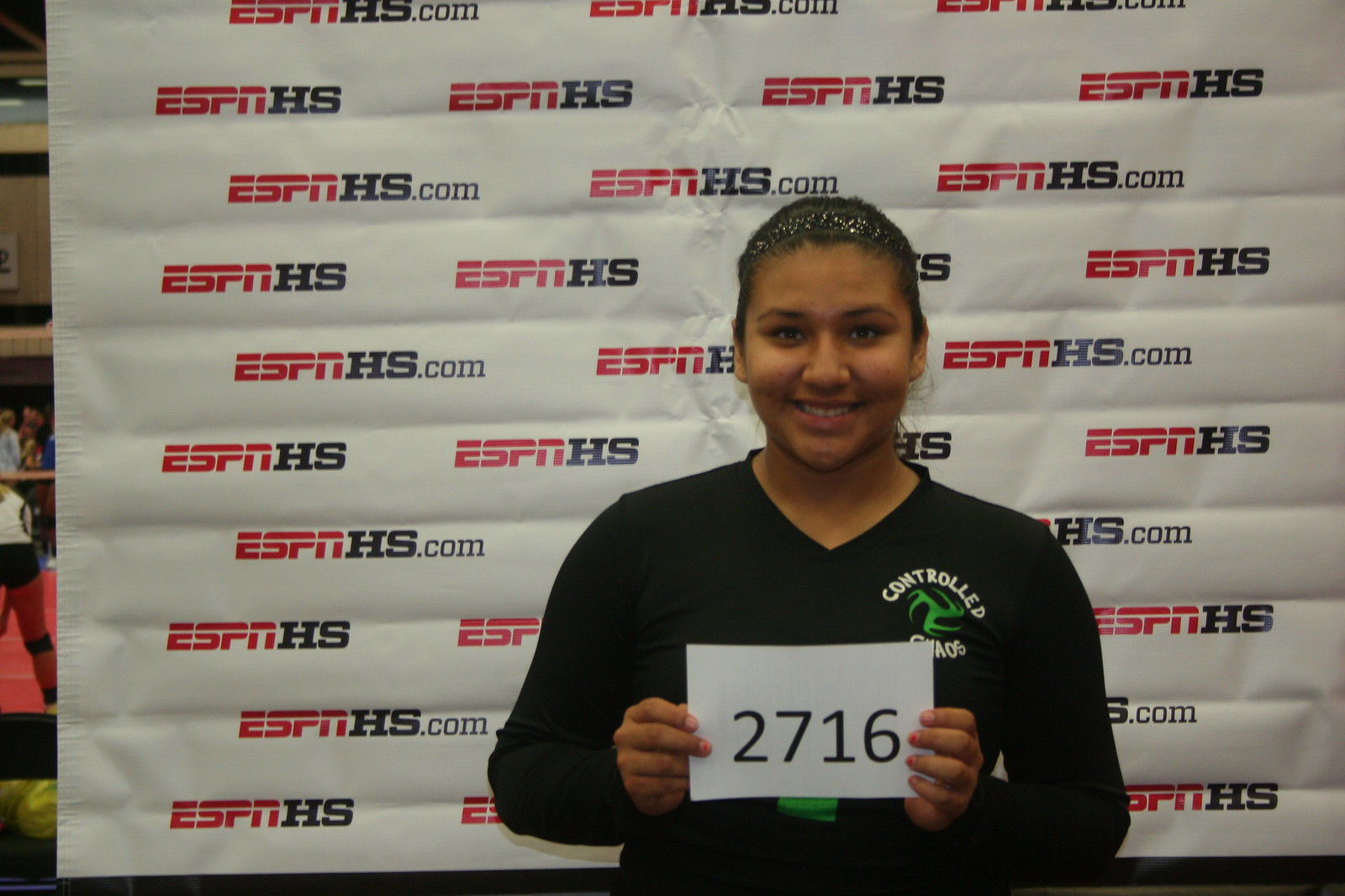The image is a photograph of a young woman, likely in her early teens, visible from the waist up. She has black hair pulled back into a ponytail and is wearing a sparkly black headband. She is smiling warmly at the camera while holding up a small rectangular white card with the number "2716" printed in black. She is dressed in a long-sleeve black shirt with a V-neck collar, featuring a white text logo that reads "Controlled Chaos" on the upper left chest, and a large green number "1" in the center. The backdrop behind her is a white banner, heavily creased in the center with multiple rows of lines indicating it is typically folded up. The banner has a repeating logo that reads "espnhs.com." The young woman radiates happiness and confidence in this engaging portrait.